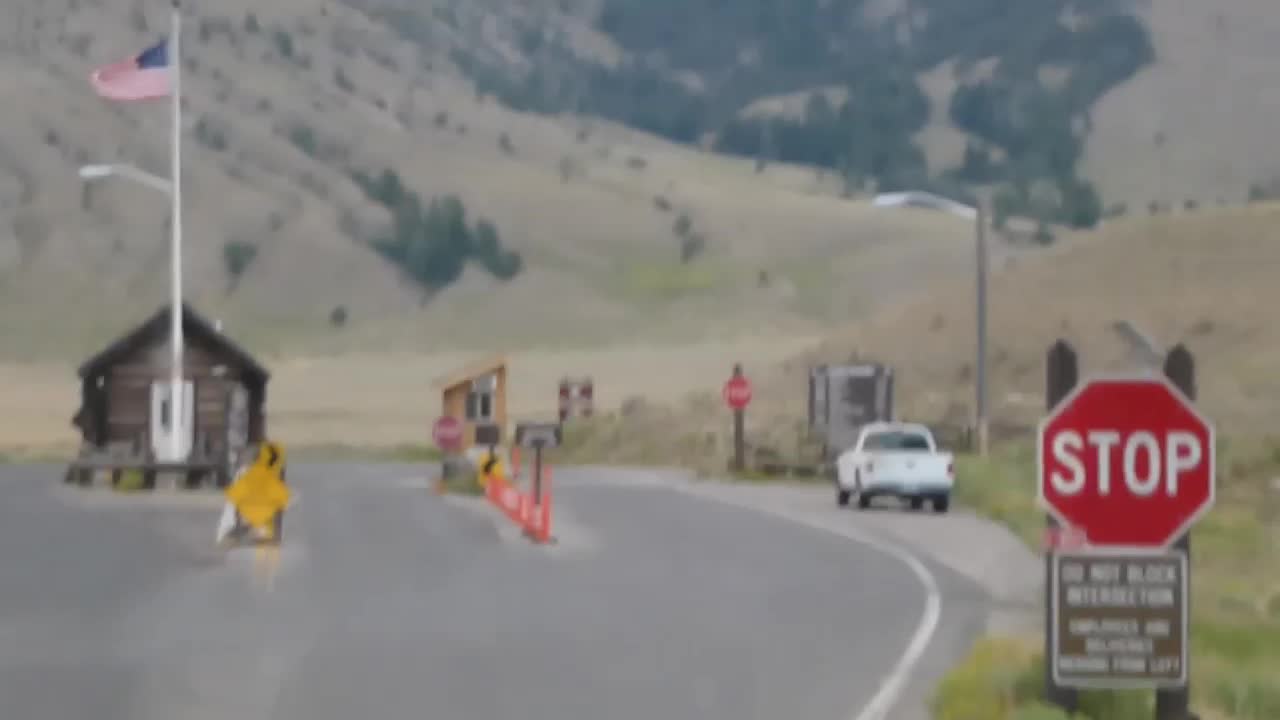This widescreen image depicts the entrance to a state park, characterized by a dual-lane checkpoint. The leftmost lane features a small wooden guard shack, equipped with an American flag mounted on a white flagpole, while the adjacent lane includes a smaller, telephone booth-sized structure. Both lanes are marked by red stop signs, with additional stop signs positioned further back. Orange cones divide the two lanes, guiding vehicles toward the checkpoint. In the forefront, a prominent red stop sign with a blurry, unreadable brown sign beneath it dominates the right side of the frame. A white vehicle is parked just before the checkpoint, yet to cross through. The backdrop reveals a vast, open valley framed by lush green hills or mountains, reinforcing the rural and picturesque setting of the park entrance.